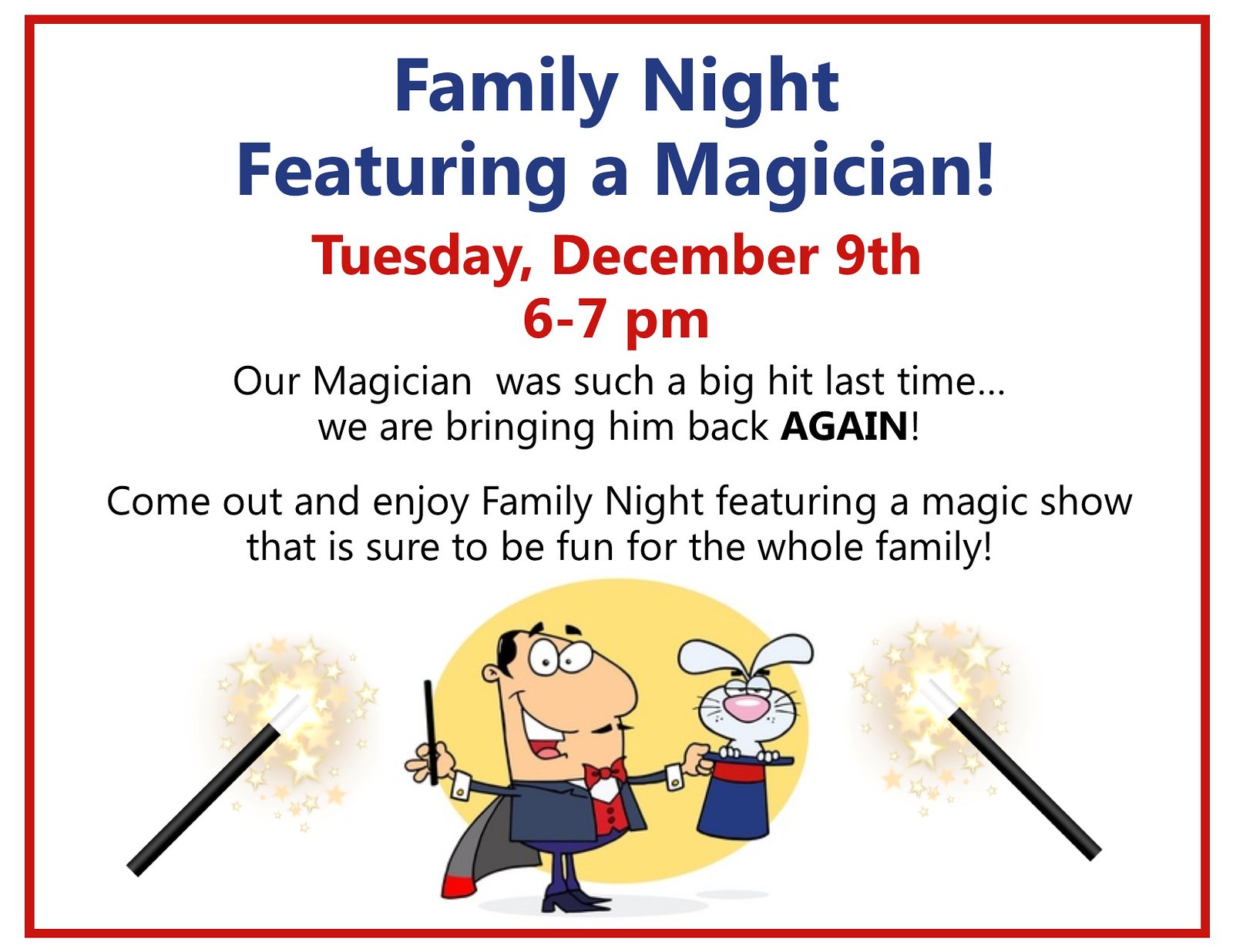The advertisement features a rectangular, slightly wider-than-tall design with a bright red border surrounding a white background. At the top, centered in bold navy blue text, it reads "Family Night featuring a Magician!" Below this, in bold red text, it states, "Tuesday, December 9th" and further down "6 to 7 p.m." In black text beneath these details, it announces, "Our magician was such a big hit last time we are bringing him back again!" Following this is an invitation: "Come out and enjoy Family Night featuring a magic show that is sure to be fun for the whole family."

At the bottom center of the advertisement, a cartoon magician is depicted. He wears a black or dark blue suit, black shoes, a black and red cape, a red vest, a white undershirt, and a red tie. He has a mustache and holds a black wand in his right hand. In his left hand, he holds a blue and red top hat from which a white bunny with a pink nose is emerging. Behind the magician and the rabbit is a yellow circle or oval, and flanking them are two black wands with white, sparkling tips. The overall imagery and vibrant colors highlight the family-friendly, magical theme of the event.